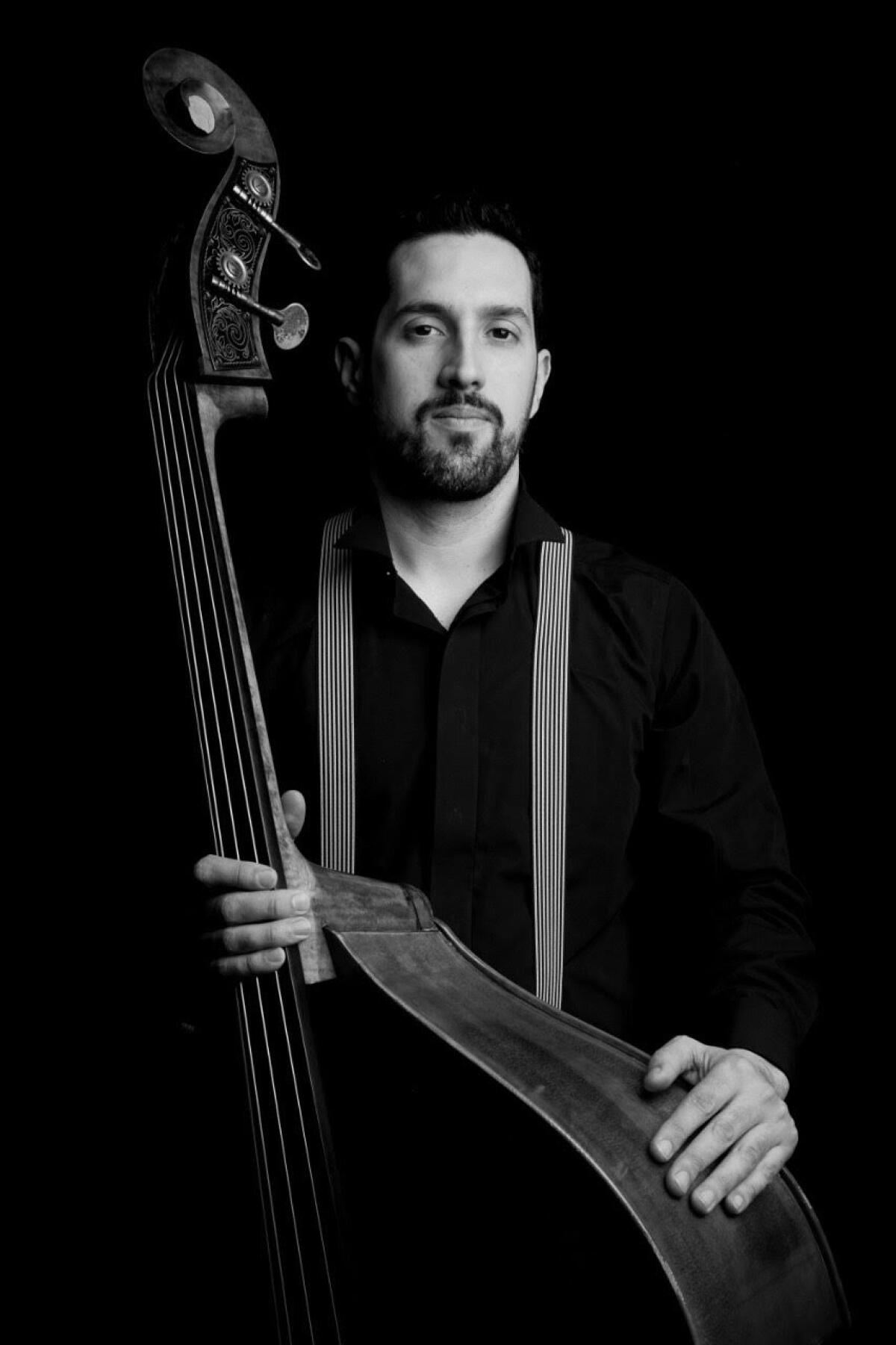This black-and-white photograph captures a Caucasian man, likely in his thirties, standing against a black background. He has dark, blackish hair, and his well-groomed goatee almost merges with his sideburns. His facial features are striking, with nicely shaped eyebrows framing an intense gaze directed at the viewer. The man sports a black, button-up, collared long-sleeve shirt and white-and-gray striped suspenders. He holds a large, unique cello that stands as tall as he does. His long fingers of one hand rest on the strings of the instrument, while the other hand grips the cello's body. The photograph exudes a relaxed yet poised demeanor, as if taken during an intimate moment between the man and his beloved instrument.